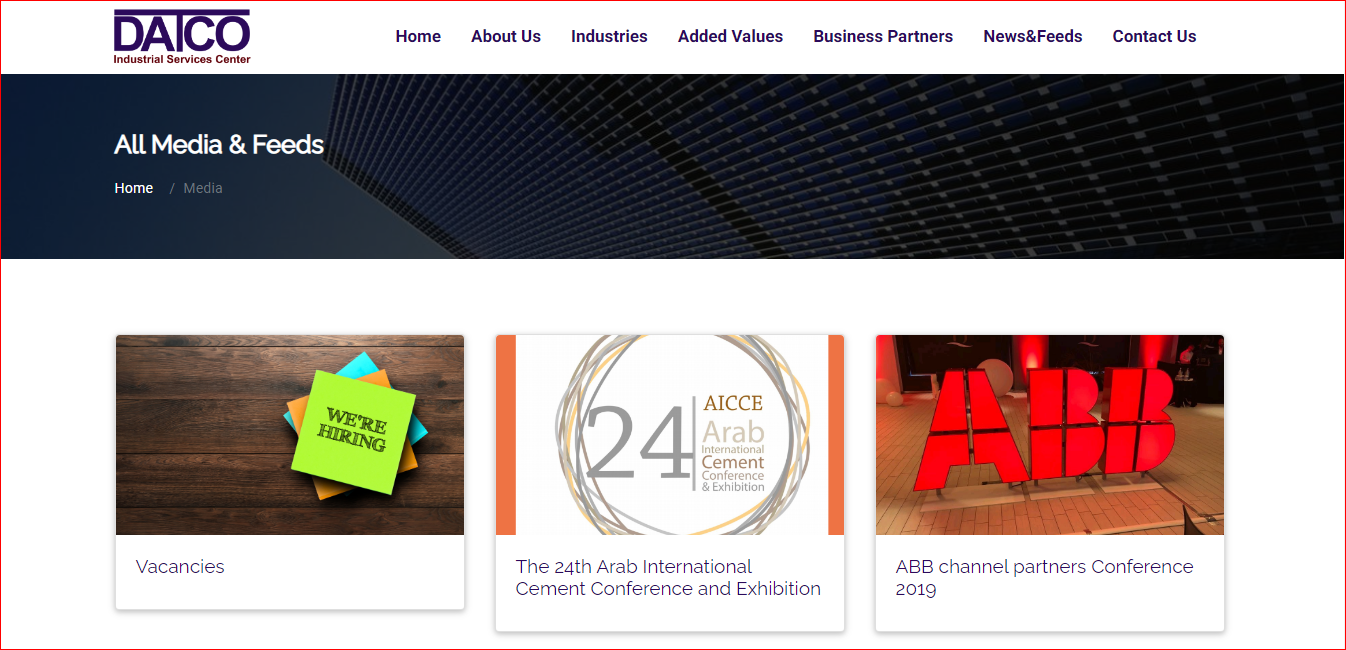This image is a detailed screenshot of the Datco website, specifically highlighting the "All Media and Feeds" section. In the top left corner, the website features the company logo with "Datco" displayed in large purple font. Directly below, in smaller red font, the text "Industrial Business Center" indicates the type of company.

To the right of the company logo, there is a navigation bar with several tabs listed from left to right: Home, About Us, Industries, Added Values, Business Partners, News and Feeds, and Contact Us. 

Below this horizontal navigation bar, there is a section header that highlights the active tab, which is "All Media and Feeds." Just beneath it, a subsection label reads "Home and Media," indicating the current subsection.

The background of this section features an image resembling a data center system. Further down, three distinct posts are displayed against a white background, each post showcasing a title and an image.

1. **Leftmost Post:**
   - **Title:** Vacancies
   - **Image:** Wooden background with post-it notes that read "We're Hiring."

2. **Middle Post:**
   - **Title:** The 24th Arab International Cement Conference in Exhibition
   - **Image:** The logo for the event.

3. **Rightmost Post:**
   - **Title:** ABB Channel Partners Conference 2019
   - **Image:** An image featuring the ABB logo.

This comprehensive view offers a clear structure of the Datco website, focusing on the "All Media and Feeds" section and its current content.